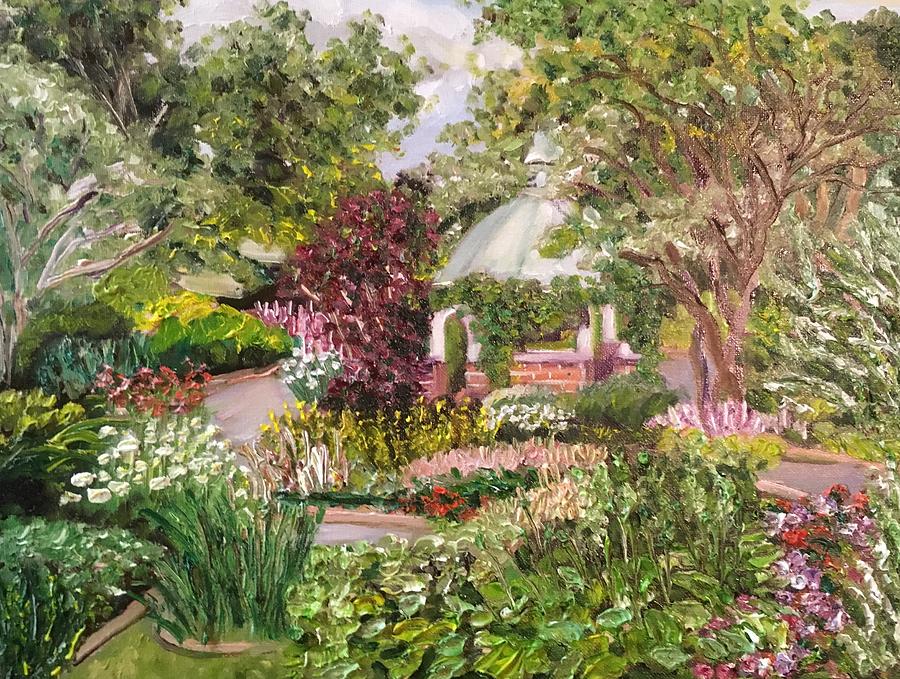In this vibrant painting, depicted in an oil paint style with an abstract touch, a lush garden or park scene unfolds, showcasing an array of detailed flora and architectural elements. Predominantly filled with greenery, the foreground is adorned with yellow, red, and purplish-red flowers alongside green bushes and possibly hostas. A striking feature in the center is a charming gazebo, identifiable by its white, vine-covered pillars and brick base, its domed roof peeking out amidst the foliage. The gazebo is surrounded by snaking paths that seem to guide the viewer through the scene. 

To the left, clusters of yellow, red, and white flowers intermingled with trees add depth, while a patch of grass claims the bottom left corner. Towards the back of the garden, amidst more trees and plants, pink flowers can be spotted. Notably, a braided tree with green and yellow leaves stands out, adding a unique touch to the scenery. On the right, another tree with yellow blooms graces the top section, contributing to the composition's balanced aesthetic. Above, a sliver of cloudy blue sky hints at the garden's open-air nature. The overall image captures the essence of a meticulously cultivated botanical paradise, inviting calm exploration and appreciation.